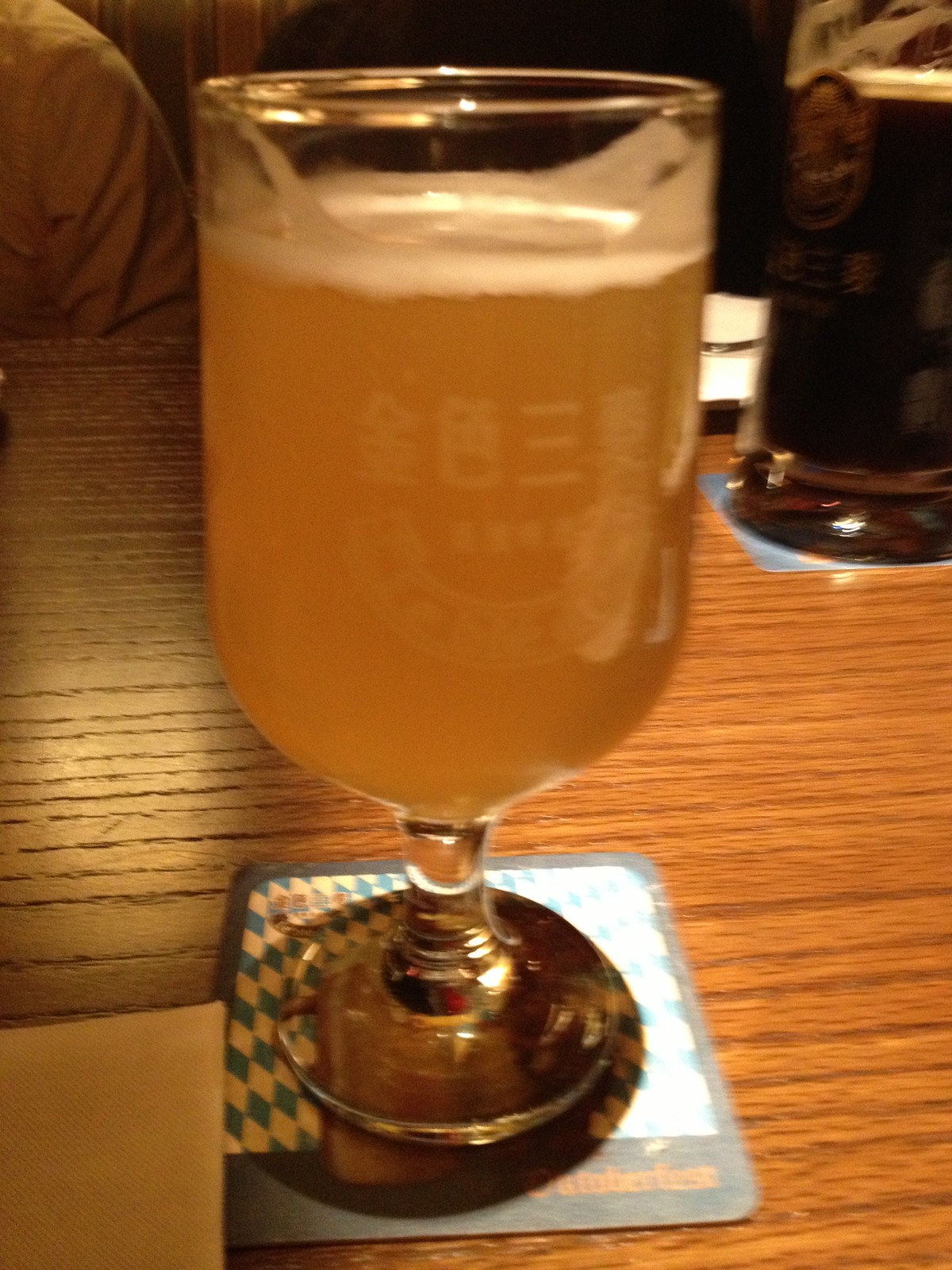A dimly lit photograph captures a neatly organized wooden table with a light blonde tone, hinting at a cozy yet refined bar atmosphere. At the forefront sits a tall, elegant goblet of amber-colored beer, nearly full with a small white head of foam. This distinctive glass, featuring stenciled writing in an East Asian script, rests upon a blue and white checker-patterned coaster branded "Oktoberfest." To the side, a napkin slightly overlaps the coaster, adding to the organized scene. In the background, a clear, tall beer stein brimming with a darker ale and a touch of foam adds depth to the image. A man's shoulder, clad in a white or light-colored shirt, is visible, suggesting he is engaged in enjoying his beer. The subdued lighting enhances the intimate ambiance, making the scene feel inviting and warm.